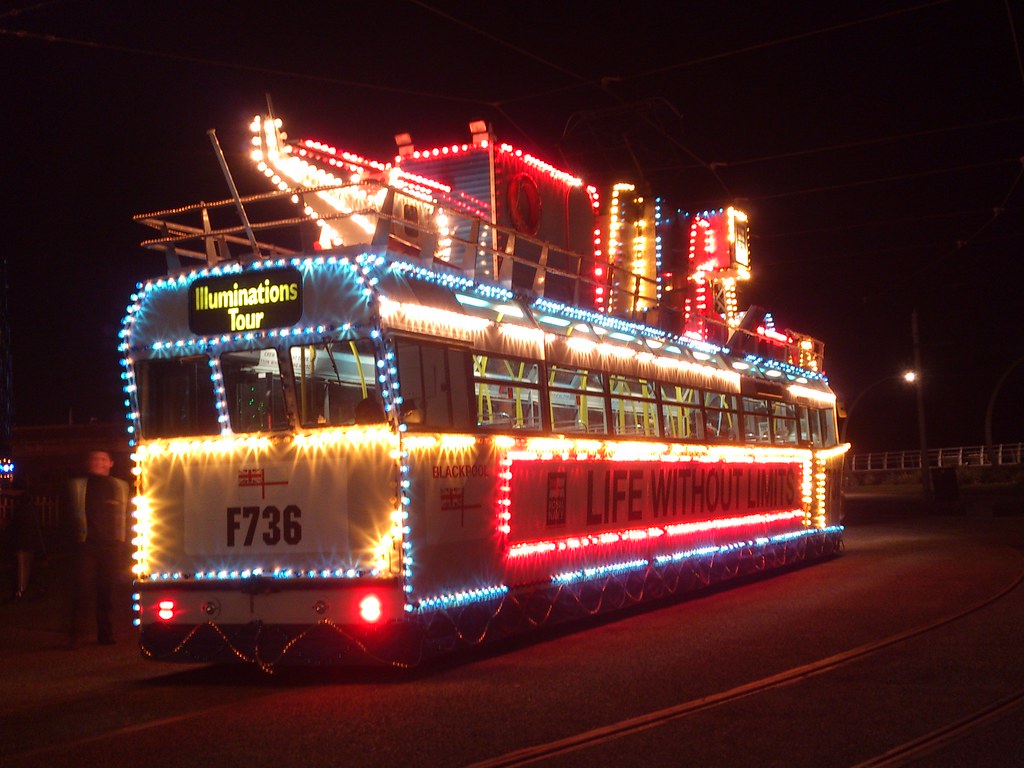In this nighttime photograph, a brightly lit and festively decorated bus is prominently featured. The front of the bus is visible on the left side of the image while the side panel extends towards the middle and right. Above the windshield area, a sign reads "Illuminations Tour," and underneath it, the code "F736" is displayed. On the right panel, a message in bold letters reads "Life Without Limits." The bus is adorned with an array of Christmas-type lights in vibrant colors including yellow, blue, red, and white. A striking row of blue lights traces the contour of the bus from the base to the top and along the back. Various illuminated objects and garlands are also positioned atop the bus, enhancing its festive appearance. The scene is set against a dark, black sky, and there are no people or other vehicles visible on the road surrounding the bus. Vertical yellow bars, meant for passengers to hold on to, are noticeable inside the bus.